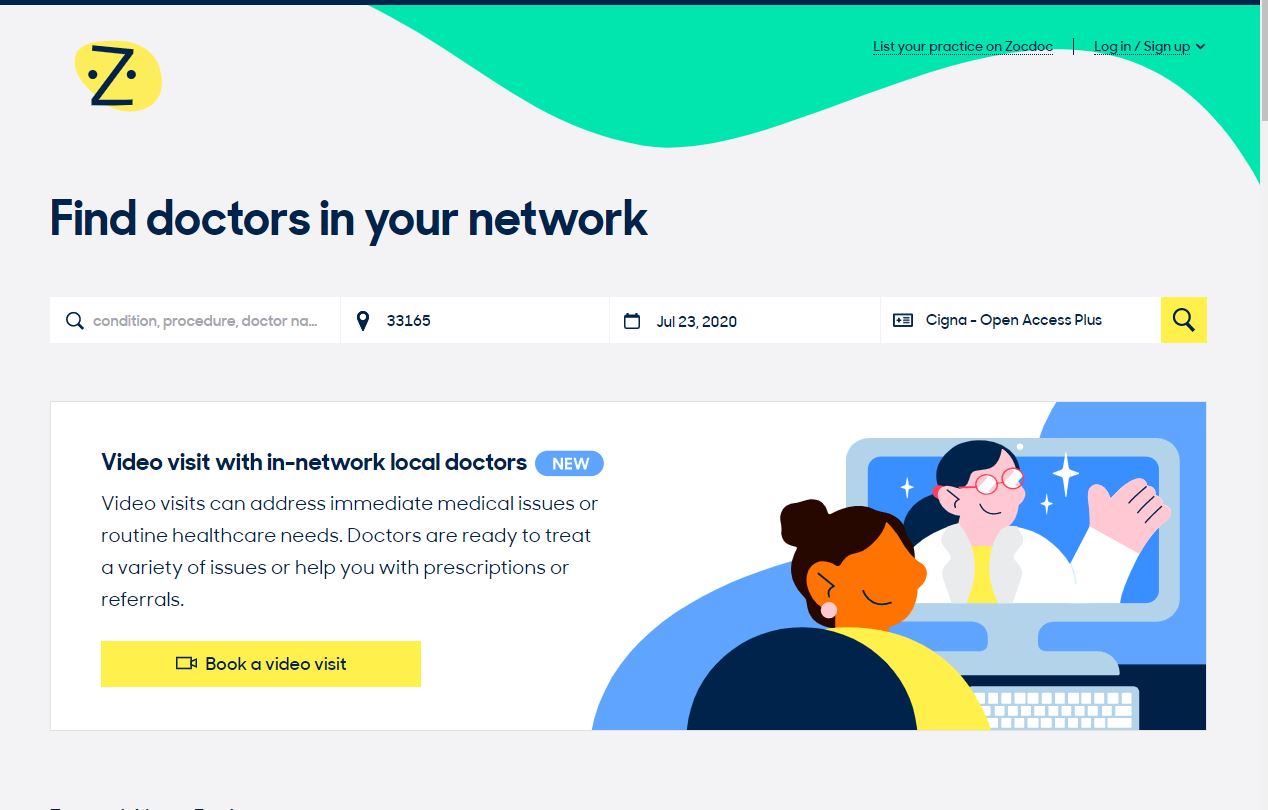The web page for the medical site features a header with an irregular yellow circle in the top left corner. Inside the circle is a large letter "Z" next to two eyes, resembling a person's face. In the top right corner, there's a prompt that reads, "List your practice on ZocDoc. Log in / Sign up."

Below this, the text "Find doctors in your network" is prominent. The first search bar is labeled "Condition, procedure, doctor," followed by another bar with the text "33165". Next to this is a bar displaying a calendar icon and the date "July 23, 2020." Adjacent to it, another bar reads "Cigna. Open Access Plus."

Further down, a section highlighted in a blue icon announces "New" features: "Video visit with in-network local doctors. Video visits can address immediate medical issues or routine health care needs. Doctors are ready to treat a variety of issues or help you with prescriptions or referrals." 

Beneath this, a yellow rectangle contains an image of a video camera alongside the text "Book a video visit." To the right of this, an image depicts a woman sitting at a desk, looking at her computer screen. On the monitor, a woman with long hair tied back in a ponytail, wearing glasses and dressed in white, is looking back at her.